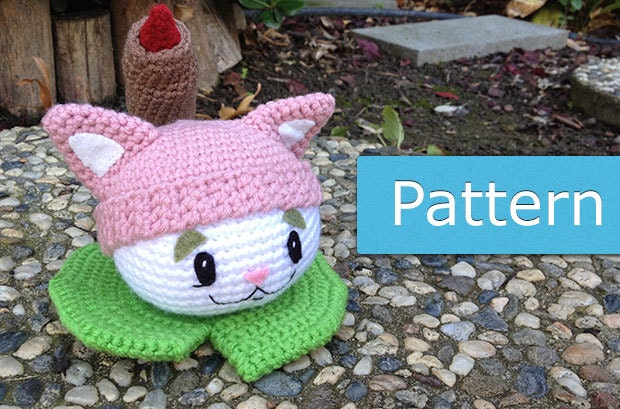In this image, the main highlight is a colorful woolen toy in the shape of a whimsical rabbit's head, lying on a rocky surface. The toy features a white face with black eyes, a green collar, and a pink and white hat with pink ears. The base color of the toy's body is green. Surrounding the toy, there are various elements that add to the scene's complexity: rocks with pebbles or mortar in between, mud, and some leaves scattered on the ground. Additionally, wooden planks and cement blocks forming steps or a walkway can be seen in the background. There is also a blue rectangle with white text on it, emphasizing the computerized look of the image.